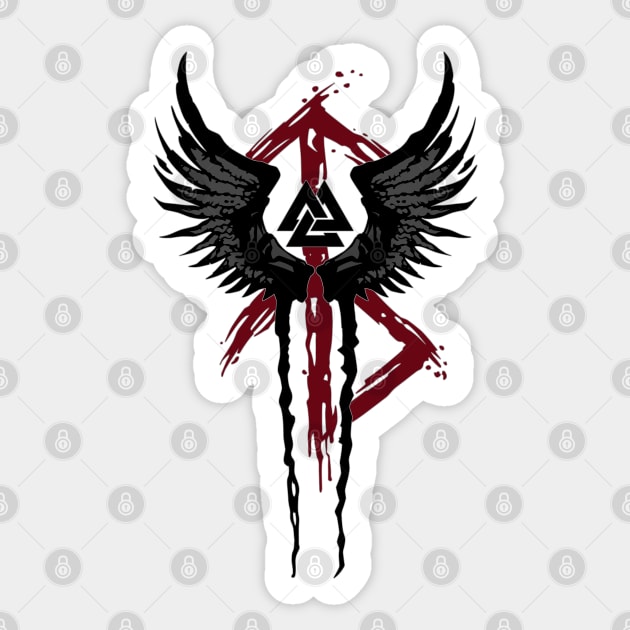The image features a stylized logo set against a light gray background, which is heavily watermarked with dark gray padlock icons arranged in a checkerboard pattern. At its core, the design showcases a pair of black and gray unfurled wings, positioned to form a prominent U shape. These wings are detailed with subtle shading to emphasize their feathering. Centrally located between the wings are three interlocking black triangles forming a continuous, interlooping path. A vivid dark red painted stripe runs vertically through the middle, extending across the top, resembling dripping paint and some splattered spots for a raw, visceral impression. From the bottom of the wings, two long, black trailing elements hang down. The entire structure is set off by a white border and drop shadow, adding depth to the logo against the light gray backdrop.